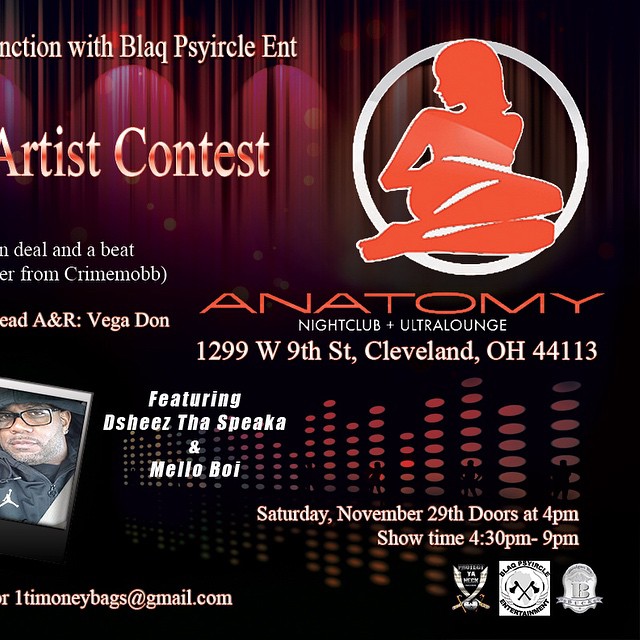This advertisement for an artist contest at Anatomy Nightclub and Ultra Lounge, located at 1299 West 9th Street, Cleveland, Ohio, 44113, features a vivid backdrop of dark red curtains. In the upper left corner, partially obscured, is "With Black Psircle Ent." Prominently displayed in a white circle on the upper right is a striking red silhouette of a woman, suggestive and artistic, with the word "Anatomy" boldly written in red beneath her. Below it reads "Nightclub and Ultra Lounge."

To the bottom left is a photograph of a black gentleman wearing a Nike jacket and glasses. Adjacent to him, the event boasts performances "featuring Da Sheez Tha Speaka and Mellow Boi." Details further disclose that the event is scheduled for Saturday, November 29th, with doors opening at 4 PM and the show running from 4:30 PM to 9 PM. Also included in the advertisement is an email address for additional information: 1timoneybags@gmail.com.